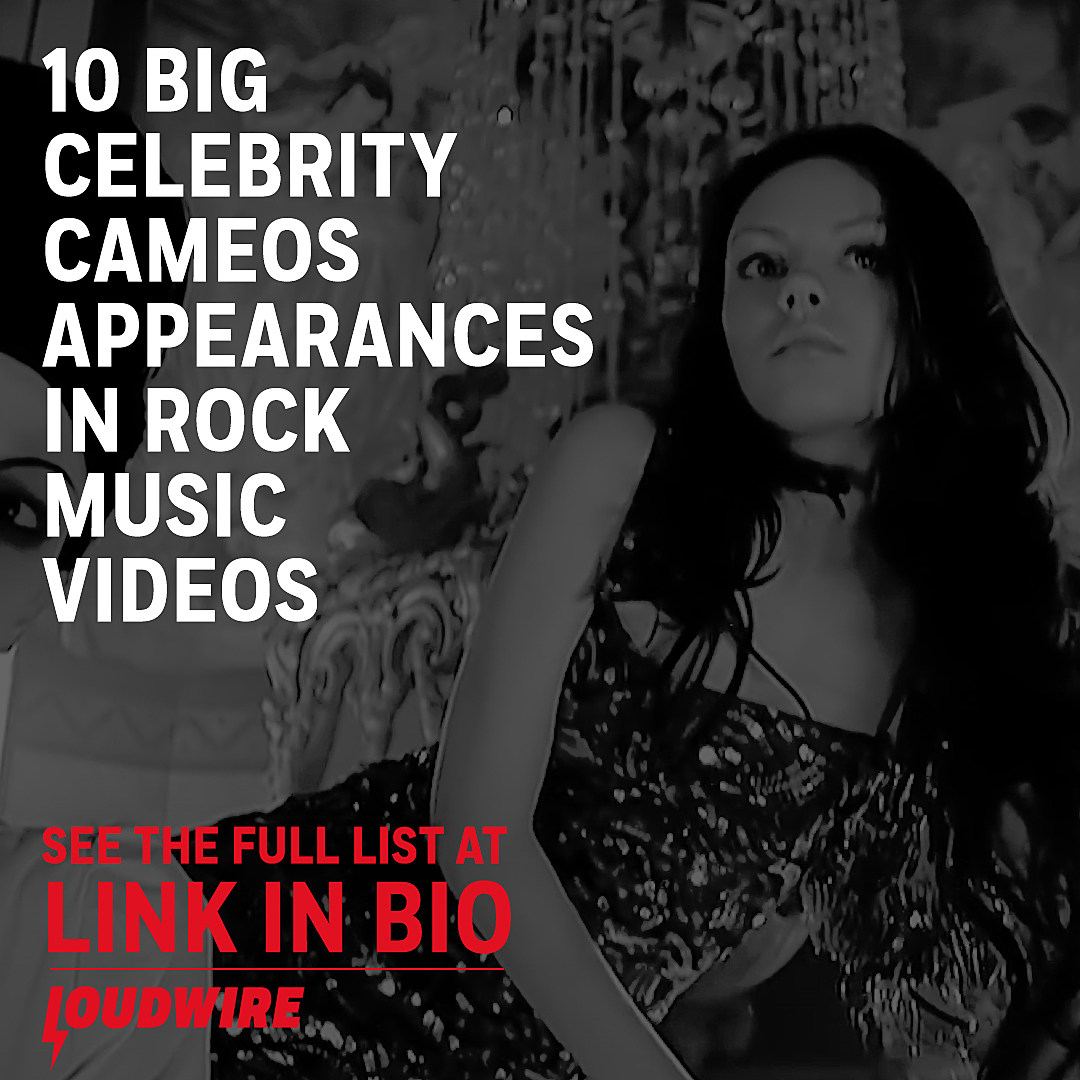A black and white advertisement image predominantly features a young Caucasian woman with long, dark, ruffled hair wearing a sequined bodysuit and a black choker. She is reclining on her side, leaning forward with her left arm in front of her, and the background is blurred but includes large crystal curtains and a column. The image is overlaid with text sections: at the top left in white letters, it reads "Ten Big Celebrity Cameos, Appearances in Rock Music Videos." At the bottom left in red text, it states "See the full list at link in bio," followed by "Loudwire," with the 'L' shaped like a lightning bolt.